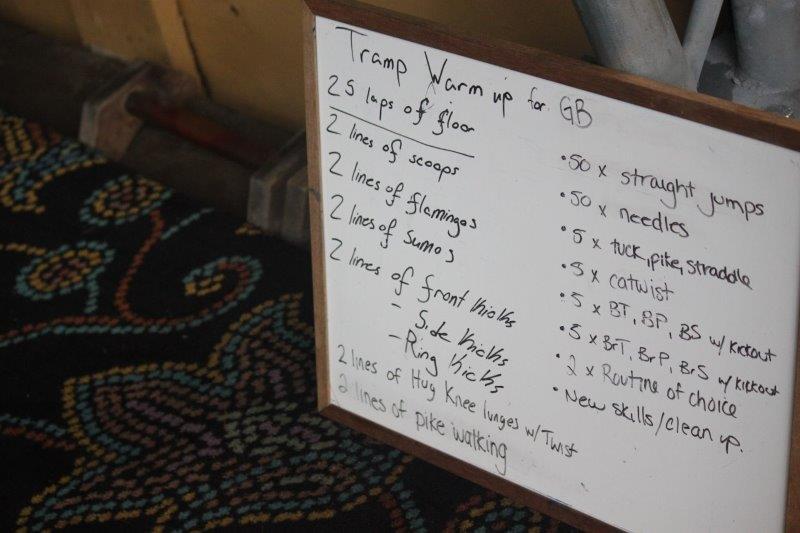The image depicts a white dry erase board with a brown wooden frame, positioned on a black carpet adorned with intricate patterns of flowers, vines, and fragmented shapes in blue, yellow, pink, and white. The whiteboard, written in black marker, displays what appears to be a detailed workout plan for a tramp warm-up session geared towards "GB." The plan meticulously outlines various exercises:

- "25 laps of floor"
- "2 lines of scoops"
- "2 lines of flamingos"
- "2 lines of sumos"
- "2 lines of front kicks, side kicks, ring kicks"
- "2 lines of hug knee lunges with twist"
- "2 lines of pike walking"

Additionally, the right side of the board lists a series of exercises to be performed in sets of 50:

- "50 straight jumps"
- "50 needles"
- "50 tuck, pike, straddle"
- "50 cat twist"
- "50 BTB PBS with kick out"
- "5 BTBRP BRS with kick out"

Finally, it concludes with instructions for "2 routines of choice" and mentions "new skills/cleanup" at the bottom. The detailed layout and structured format clearly highlight this as a comprehensive workout agenda.